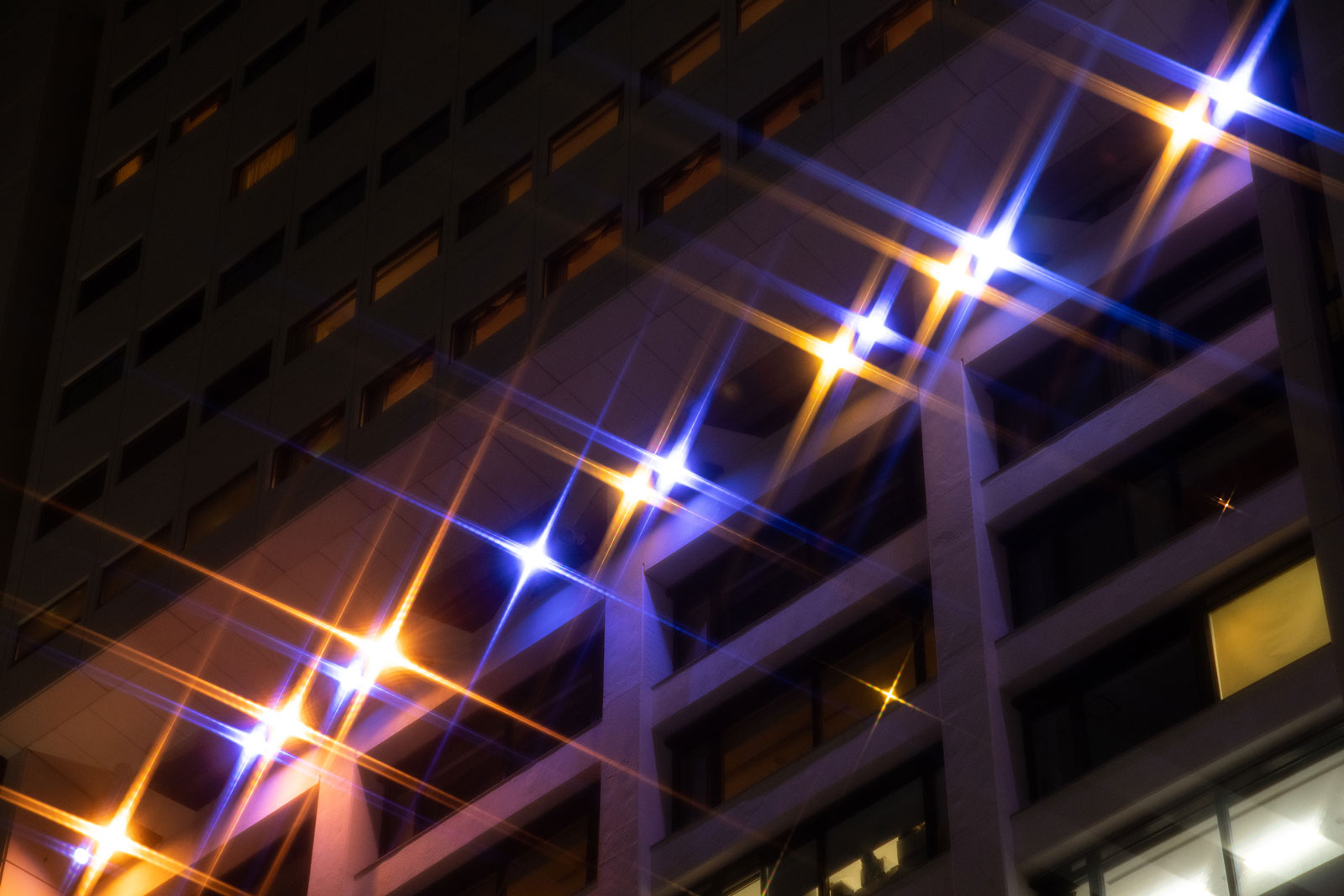The image captures a tall apartment building, photographed at night from a low angle, looking up. The building's facade is divided into two main sections: the upper part is colored gray and houses many smaller windows, while the lower part is white with larger windows. The focal point of the image is a series of alternating blue and orange-yellow lights situated in the middle of the building, just above a ledge. These lights cast striking X-shaped patterns due to overexposure. The dark night sky serves as a backdrop, enhancing the contrast of the building's illuminated and dimmed windows. The overall scene is detailed and dramatic, emphasizing the building's height and the interplay of light and darkness.